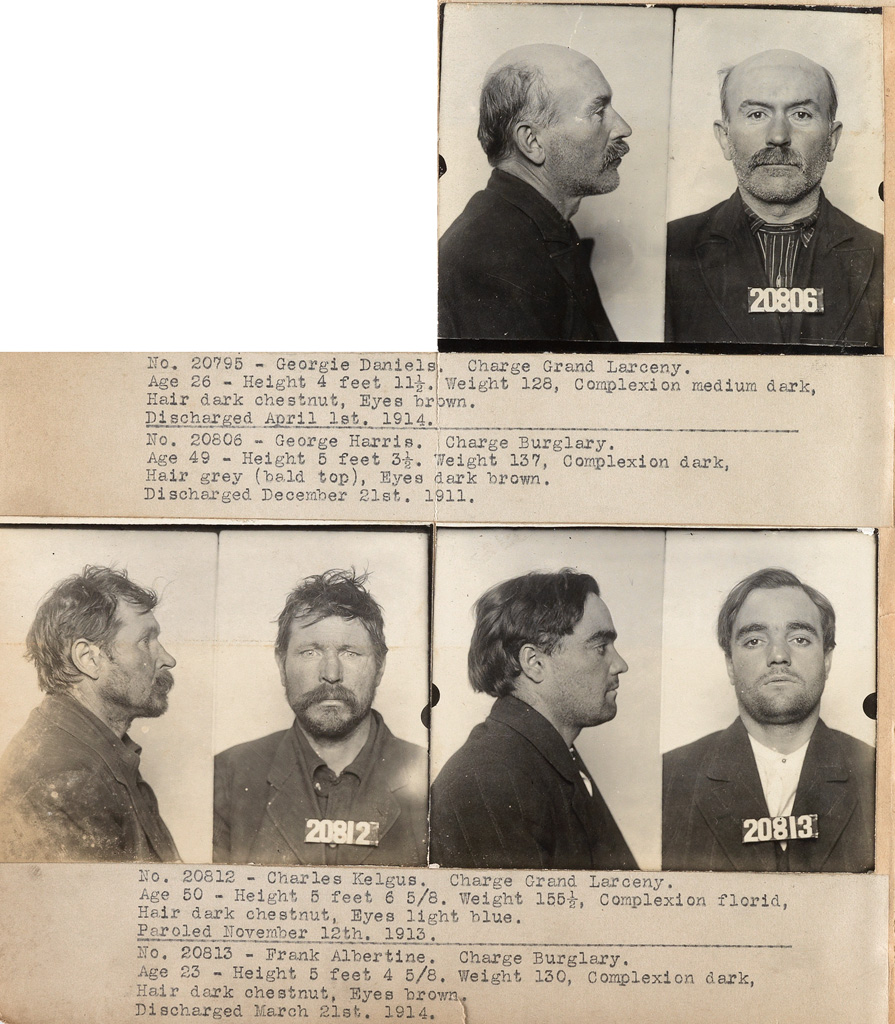The image is a black and white poster showcasing a series of mugshots from around the early 1910s. The poster features six mugshots in total, with two images of each man: one from the front and one in profile. At the top, there is a bald man with a mustache, identified by prisoner number 20806. The text below his mugshots, partially missing and too small to fully read, indicates his name and charges—though part of it has been obscured, it can be inferred that he was involved in criminal activity. 

In the lower part of the poster, there are two additional men. The first, under prisoner number 20812, is Charles Kelg, charged with grand larceny. He has disheveled hair and a brown beard and mustache. Next to him, under prisoner number 20813, is Frank Abertine, charged with burglary. He has combed brown hair, a short five o'clock shadow, and bushy eyebrows.

The poster appears old and worn, with faded ink and missing sections, and it possibly dates to between 1911 and 1914. The document's vintage nature is hinted at by a slightly pinkish hue in the paper and the deteriorating condition of the images.